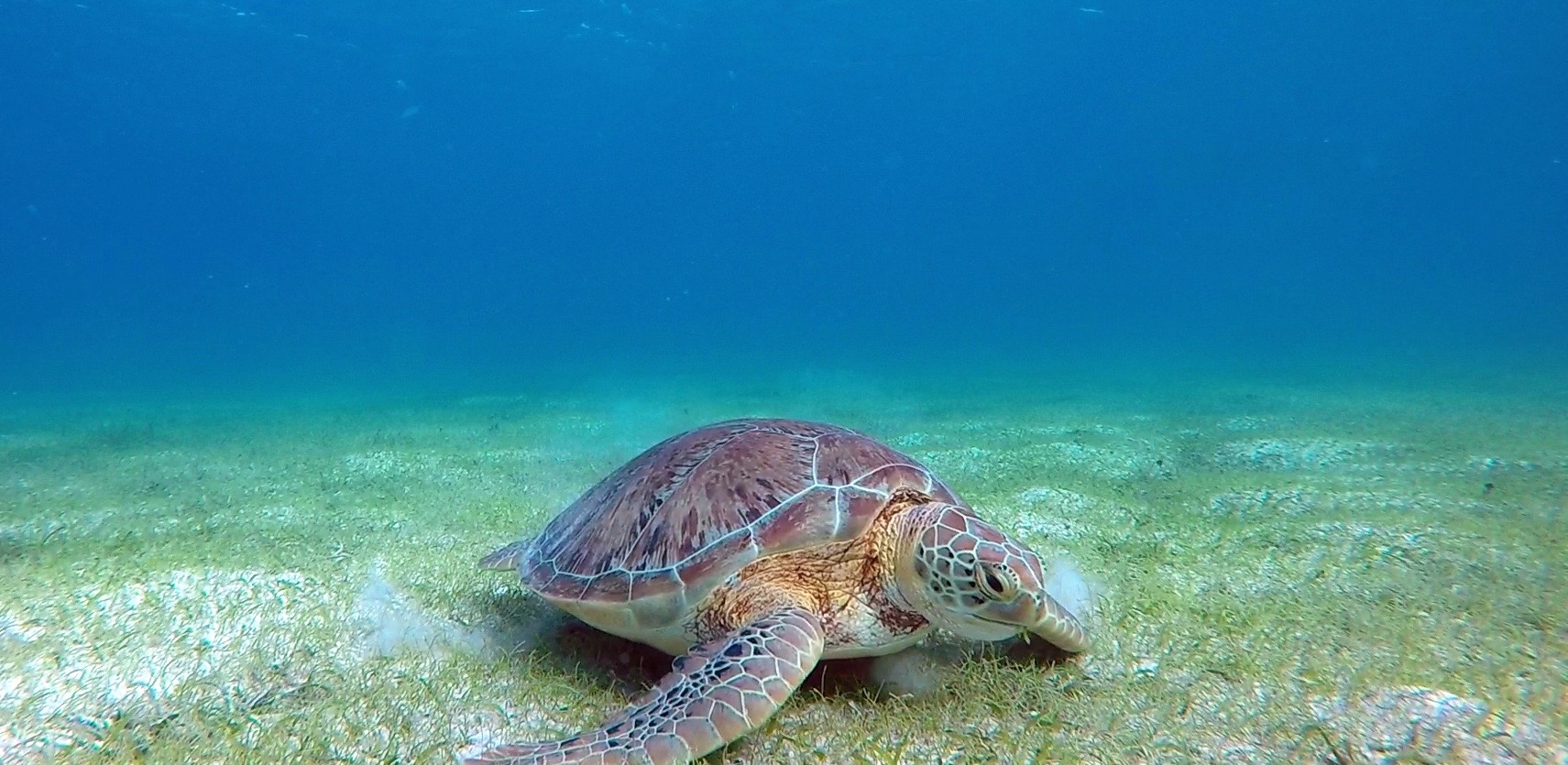In this captivating underwater scene, a sea turtle rests peacefully on the seafloor, surrounded by the vibrant colors and textures of a shallow ocean bed. The turtle, positioned towards the bottom middle of the image and making its way towards the bottom right, features a mottled gray shell with patches illuminated by the water's blue and green hues. Its large flippers are poised, suggesting a moment of calm amidst subtle underwater currents. The surrounding seafloor is a canvas of lightly covered green vegetation and faintly visible white sand, punctuated by small grasses and plants. The background extends into deeper shades of ocean blue, creating a serene and natural underwater tableau.